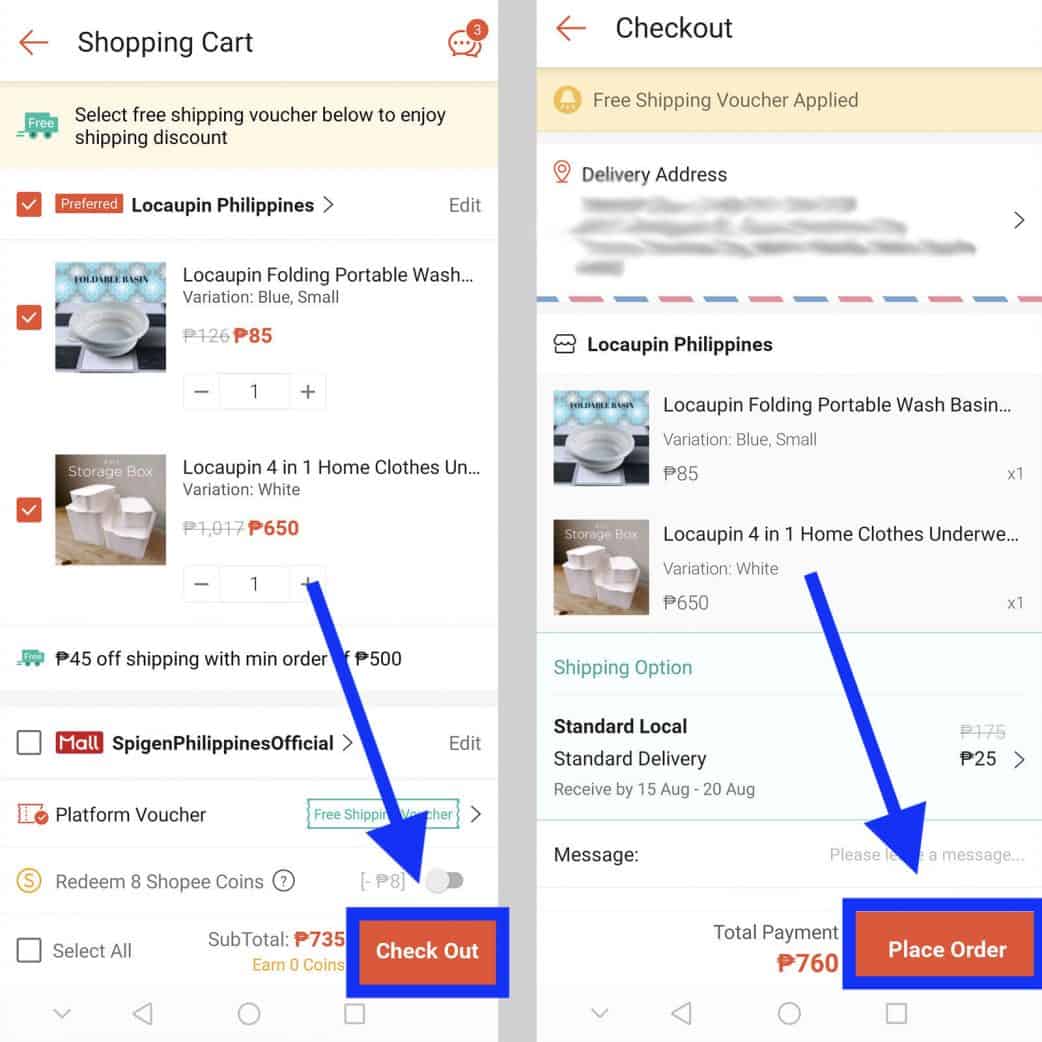This image consists of two screenshots displaying different sections of a shopping experience. The left screenshot shows a shopping cart, while the right one shows the checkout page. Both headers, "shopping cart" and "checkout," are in black font. In the top left corner of each screenshot, red arrows pointing left are visible.

In the first screenshot (left side), a beige banner at the top of the screen has black text that reads "Select free shipping voucher below to enjoy shipping discount," accompanied by a green truck icon with the word "free" on it. Directly below the banner, the text "Laquapin Philippines" is displayed, with a gray "edit" button on the right. There is also a red box with a white check mark to the left.

Further down, a red rectangle with white text says "preferred." Below this, the text "Laquapin folding portable wash, variation blue small" is displayed, with another red box containing a white check mark on the left side. Adjacent to the text is an image of the said item.

In both screenshots, a chat icon with a notification circle showing the number three is positioned on the right side near the top.